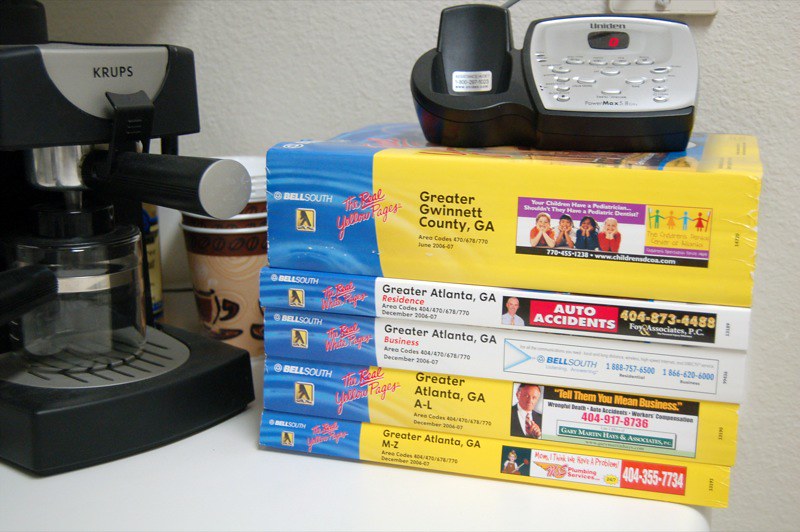The photograph features a nostalgic scene centered around a stack of old phone books prominently displayed on what appears to be a kitchen counter or a white shelf. The main focal point is the five stacked Bell South phone books, all from the Atlanta area in Georgia. The top and bottom phone books, distinctly yellow, are traditional Yellow Pages. The topmost one specifically notes 'Greater Gwinnett County,' while the bottom two are divided alphabetically into 'Greater Atlanta A to L' and 'M to Z.' Sandwiched between these are two thinner, white-bound directories—one labeled 'residential' and the other 'business' for Greater Atlanta, Georgia. Atop this stack rests an old-school landline phone base, complete with a digital answering machine display indicating zero messages. Positioning to the left of the photo is a Krups espresso maker, accompanied by a small stack of reusable paper coffee cups with lids, adding a touch of everyday life to the composition. The juxtaposition of the retro phone books and the landline phone with the modern coffee setup evokes a blend of past and present.